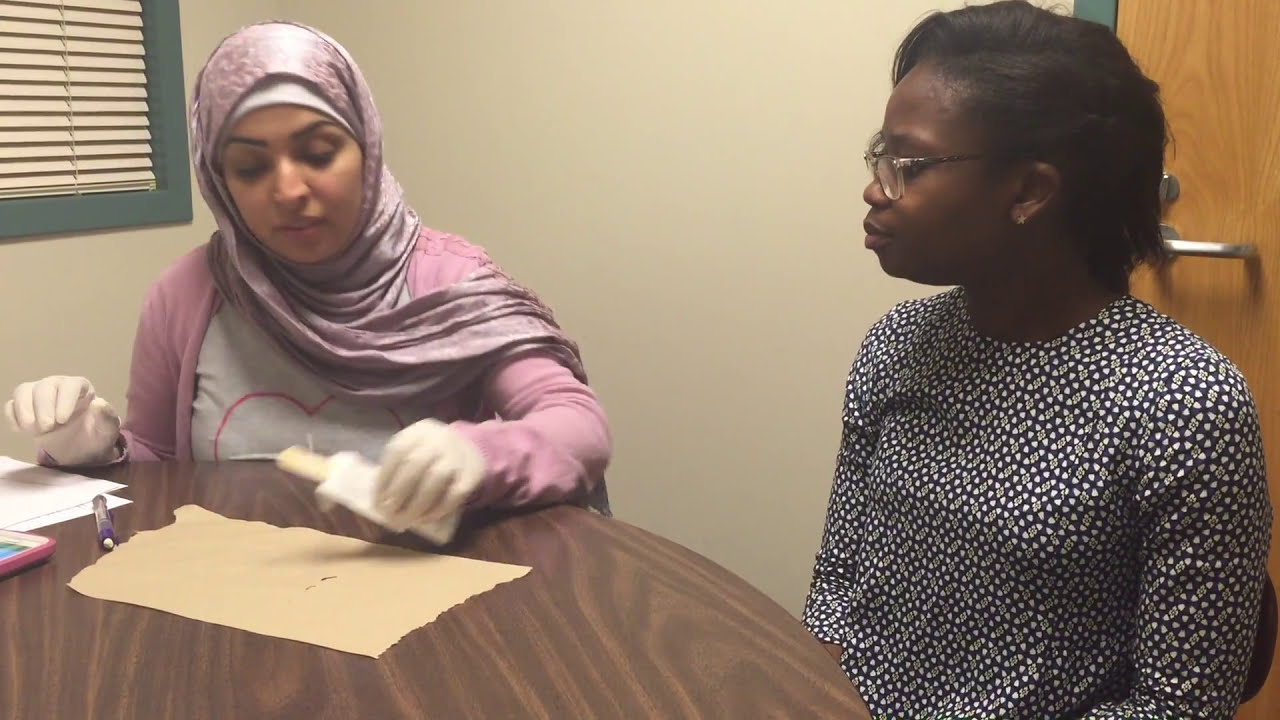The image showcases two women seated side-by-side at a dark wooden table, seemingly engaged in an educational demonstration or a collaborative activity. On the left is a woman with light brown skin, wearing a pink hijab and matching sweater over a white t-shirt that has an outline of a heart on it. She is adorned in white gloves, suggesting she is handling something delicate or conducting an experiment. Her left hand is caught in motion, slightly blurry as she appears to be pouring or placing an object onto a brown piece of paper or paper towel spread on the table. Her right hand rests on the edge of the table, fingers slightly curved. To her left lies a pencil, a cell phone, and some scraps of paper. 

Seated on the right is an African-American woman with short black hair extending just above her shoulders. She wears glasses and a blue-and-white patterned shirt adorned with circles and arrows. She is observing the woman on the left intently, indicating her active participation or interest in the ongoing activity.

The room around them is small, with white walls. To the left of the image, there is a window framed in green with white blinds partially drawn. On the right side, a wooden door with a golden brown finish, green frame, and a silver handle is visible. This detailed context and the described elements convey a focused scene that combines both educational intent and interactive engagement.